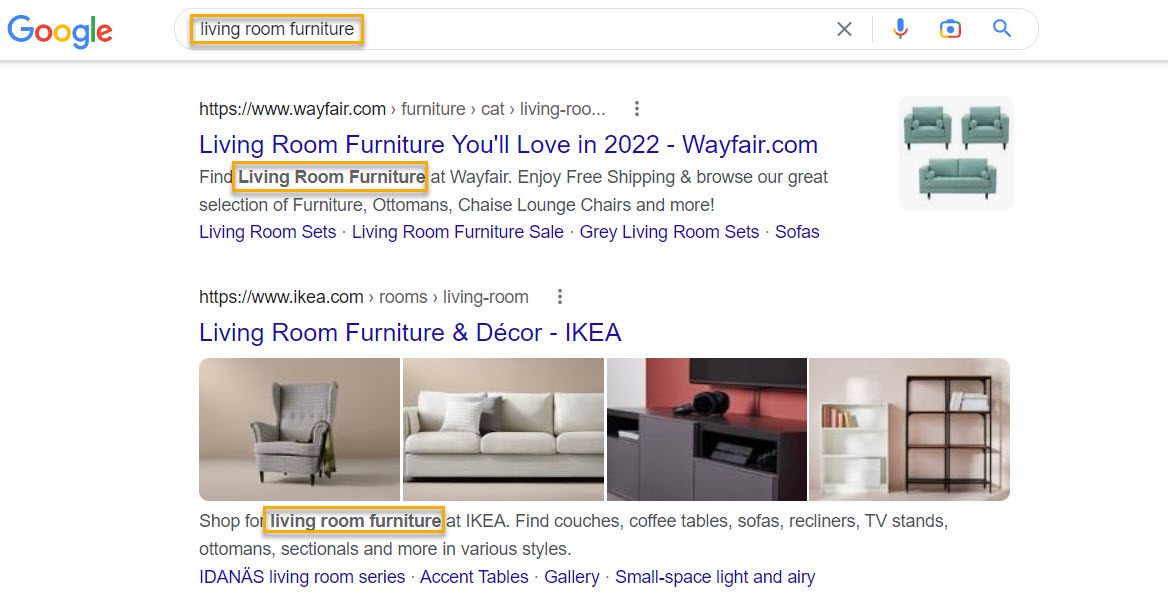This image is a screenshot captured from a desktop or laptop computer, showcasing a widescreen display. The screenshot depicts a Google search page with the iconic Google logo, adorned in its distinctive colors of blue, red, yellow, and green, positioned in the upper left-hand corner. At the very top, the search bar is clearly visible with the term "living room furniture" entered into it, emphasized by a gold-colored highlight around the text. 

Beneath the search bar, the screen reveals the search results. The view is slightly scrolled down, obscuring the options for different types of searches, such as Shopping or Images. The first visible search result is for the website Wayfair.com. The clickable link reads "living room furniture 11-20-22 Wayfair.com". Directly below this, a brief description states, "Find living room furniture at Wayfair," with the phrase "living room furniture" highlighted in the same gold box as seen in the search bar.

The subsequent search result is for IKEA, where the text "living room furniture" is likewise highlighted in a gold box within the description, ensuring consistency in the emphasis of the search term throughout the visible search results.